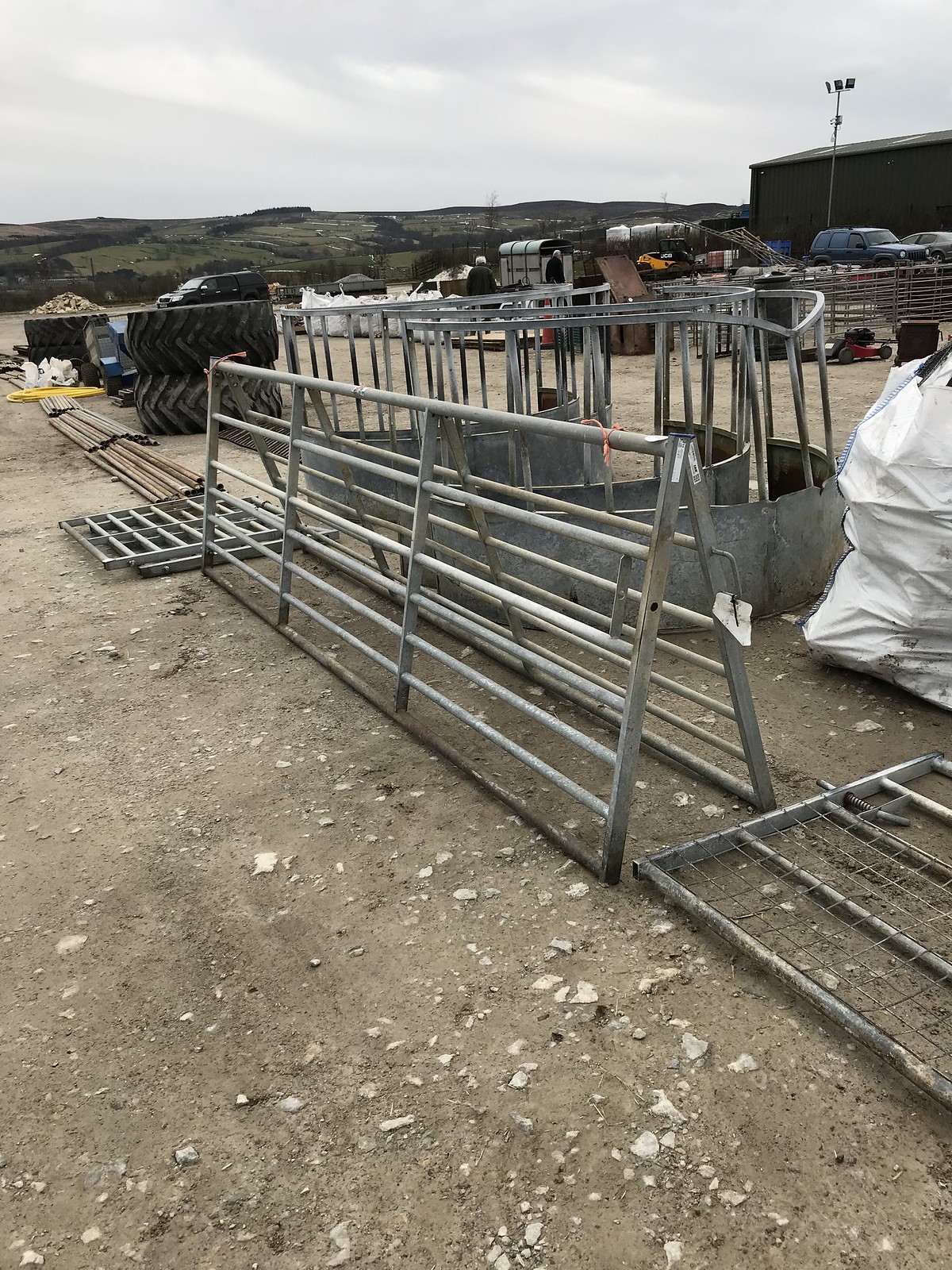The photograph depicts an outdoor industrial yard, characterized by a flat, sandy ground scattered with rocks. Dominating the foreground are a series of metal cattle fence panels, arranged diagonally from the lower right to the upper left. These panels appear to be used for setting up a rodeo or cattle operation. To the upper left of the image, two large tractor tires are visible, one stacked on top of the other, with an additional tire situated behind them. The background features gentle hills covered in patches of greenery under a cloudy sky. In this area, a variety of industrial items are scattered, including a trailer possibly for carrying gravel, piles of pipes, and several parked cars. A large brown building stands to the right, equipped with a giant pole that may hold either speakers or lights. A large, white bag, potentially for garbage, is also visible in the upper right section of the image.